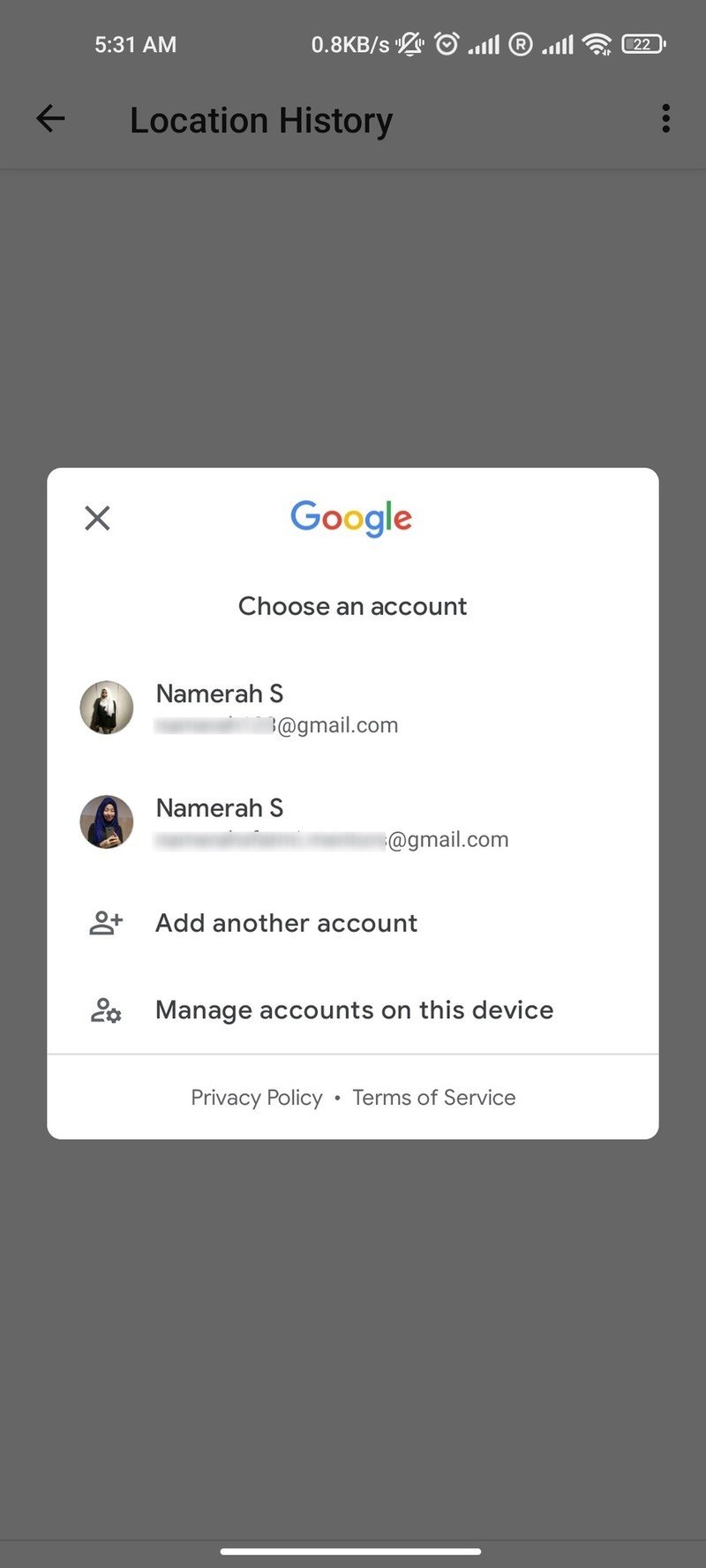This screenshot captures a smartphone displaying a Google app interface. It was taken at 5:31 AM, as indicated at the top of the phone, which also shows a data transfer rate of 0.8 kilobytes per second. The notification bell icon with a slash indicates that notifications are silenced. An alarm clock icon beside it shows that an alarm is set. The phone has full cellular service, with five signal bars and an 'R' to the right of them, indicating roaming. There's also a full Wi-Fi signal and a battery icon displaying a 22% charge.

The main content of the screenshot displays a Google app screen, which appears to be trying to access the user's location history, partially visible in the background. A dark gray overlay covers this, bringing up a white dialog box featuring the Google logo at the top with a dark gray X in the top left corner. The box prompts the user to choose a Google account to proceed. Two accounts are listed, both belonging to a user named Numera S. Namera. Their email addresses are partially obscured, leaving only the @gmail.com suffix visible. The two accounts have different profile pictures. Additionally, there are options to add another account or manage accounts on the device. At the bottom of the dialog box, links to the Privacy Policy and Terms of Service are provided.